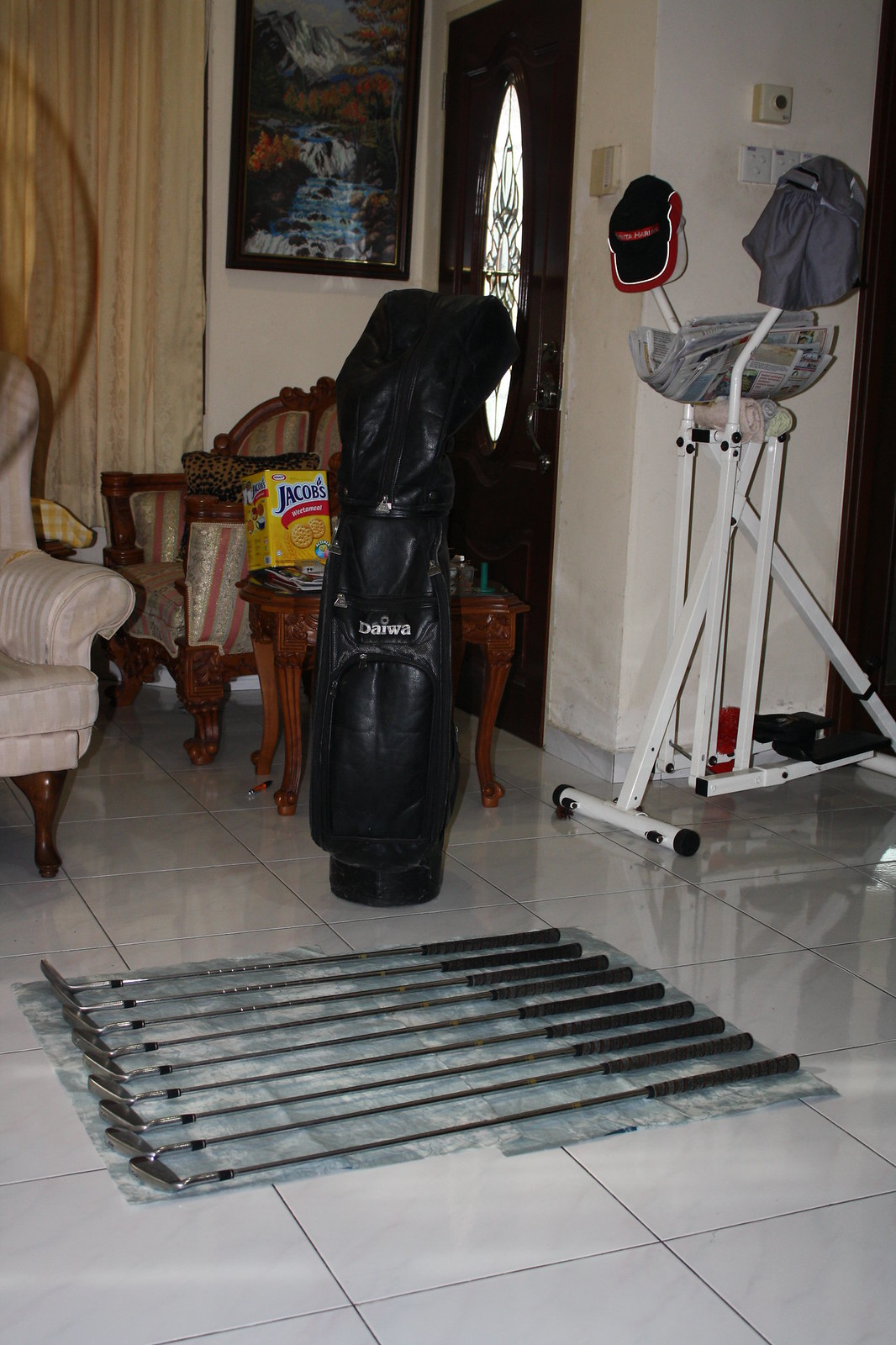This vertically oriented color photograph depicts a living room scene filled with a variety of items, focusing largely on an arrangement of golf equipment. The shiny white or gray tiled floor serves as the backdrop for a light greenish-blue piece of fabric that lies in the foreground. Neatly arranged diagonally on this fabric are eight to nine golf clubs, each appearing very similar to the next. Behind the clubs stands a tall, black, possibly leather golf bag ready to hold them. To the left, part of an ornate upholstered chair with wooden legs is visible, adding a touch of elegance to the room. On the right side, a white exercise machine is cluttered with several objects, including a baseball hat on one handle and newspapers stacked on the seat. There's also a piece of fabric draped over another handle. In the background, a wooden table holds a distinctive yellow box labeled "Jacobs." To the back, a dark wooden door with an oval-shaped window stands near a full-length yellow curtain, and adjacent to it is a wall-mounted painting of a waterfall or stream. Various knick-knacks on a coffee table add to the homely disarray of the room.